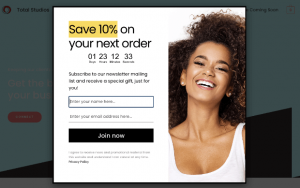The image is a screenshot of a website that has been partially grayed out, with a pop-up advertisement dominating the page. The pop-up is a white rectangular overlay, divided vertically into two sections.

On the right side of the pop-up, there's a high-resolution image of a dark-skinned woman with long brown hair, captured from her chest to just above her head. She is wearing a white tank top and is standing against a pristine white background. Her expression is joyful, with a bright smile and a hint of laughter, exuding a sense of happiness and approachability.

The left side of the pop-up contains a promotional offer. At the top, large black text reads "Save 10% on your next order," with the phrase "Save 10%" prominently highlighted in yellow. Below this enticing offer is a countdown timer displaying "1:23:12:33," tracking the number of days, hours, minutes, and seconds remaining to avail the deal.

Following the countdown timer is a brief blurb of text, likely providing additional details about the promotion. Beneath this text, there are two input fields for the user to enter their name and email address, encouraging engagement with the offer. At the bottom of the form is a black rectangular button with the text "Join Now," inviting users to take immediate action. Below this button, there's some fine print containing promotional terms and conditions.

The overall layout of the pop-up is clean and visually appealing, designed to attract attention and encourage users to participate in the promotional offer.